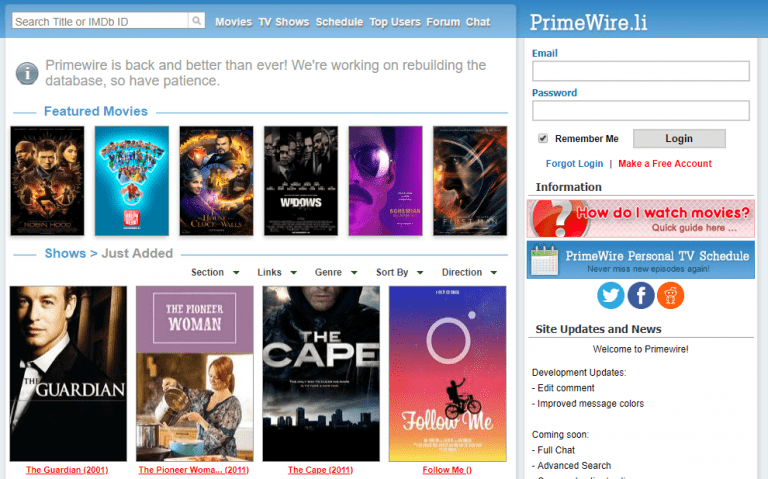The image showcases the homepage of the website primewire.li, which appears to be a platform for streaming movies and TV shows, possibly associated with piracy based on context.

At the very top left is a search bar labeled "Search title or IMDb ID." Next to it are navigation options including "Movies," "TV Shows," "Schedule," "Top Users," "Forum," and "Chat."

On the upper right-hand side, there are fields for "Email" and "Password," both highlighted in blue. Below these fields is a checkbox labeled "Remember me," followed by a gray "Login" button with black text. There are also links for "Forgot login?" in blue, and "Make a free account" in red.

Beneath this navigation area is informational content including a "How do I watch movies? Quick guide here" link, marked by a small red question mark icon. Additionally, there is a promotional line that reads, "Primewire Personal TV Schedule: Never miss new episodes again," accompanied by icons for Twitter, Reddit, and Facebook for social media integration.

Further down, site updates and news are listed. These include a welcome message, development updates, and notifications of new features such as "Improved message color," "Full chat," and "Advanced search." The most prominent update states, "Primewire is back and better than ever. We are working on rebuilding the database, so have patience."

Below the updates, the site displays a selection of movies, with titles like "Widows," "The Guardian," "The Pioneer Woman," "The Cape," and "Follow Me."